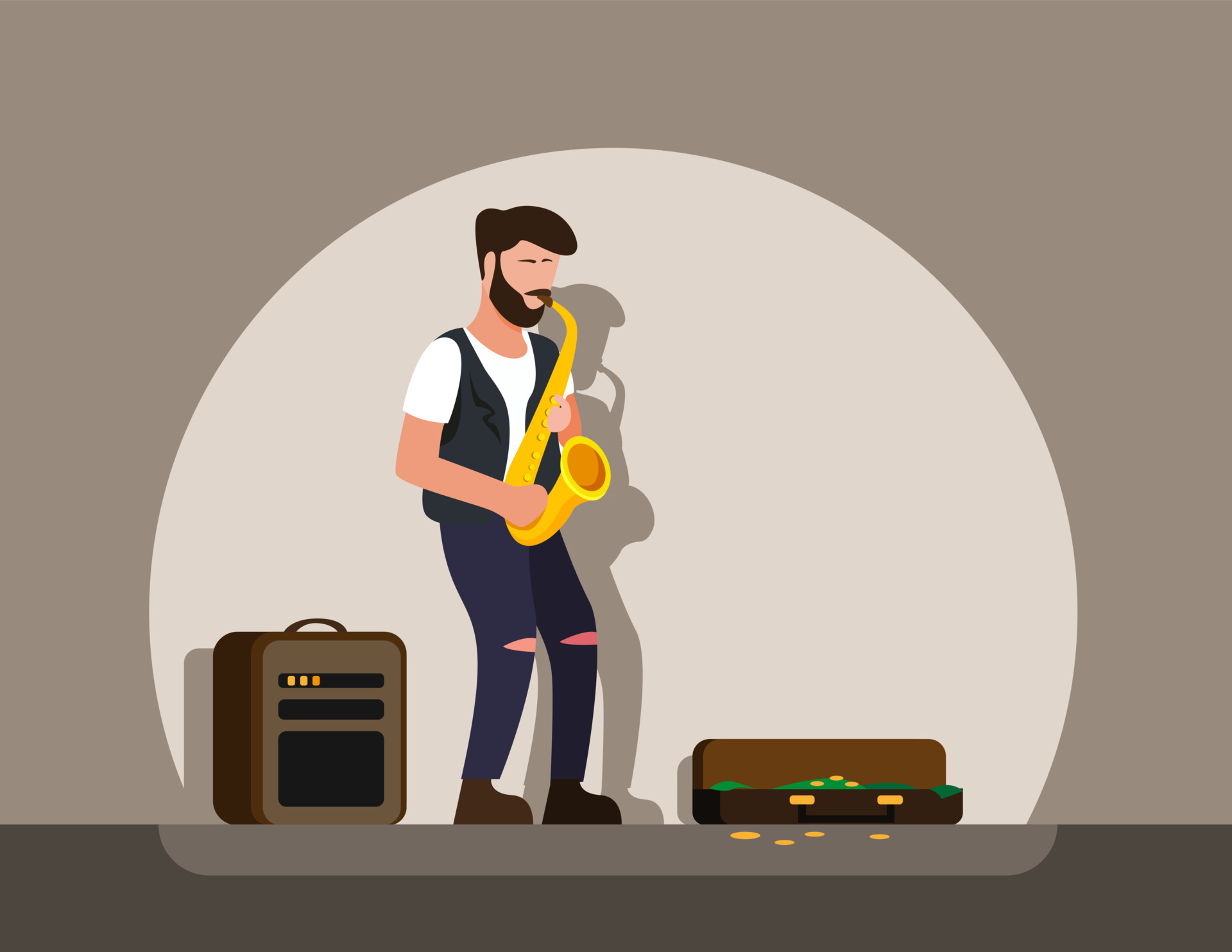In this image, we see a detailed, clip-art-style animation of a street musician busking against a tan wall, playing a golden trombone or horn instrument. The musician is a white male with short brown hair and a brown beard, dressed in blue pants with torn knees, a white t-shirt, and a dark gray sleeveless vest. He is wearing brown boots. The spotlight effect casts a semicircular white glow around him, highlighting his shadow on the wall and the darker gray ground beneath him.

To the musician's left, there is a brown speaker or amplifier with a black grille and face, adorned with yellow and orange lights and a handle on top. To his right on the ground is the open case for his instrument, which is brown with gold latches and filled with gold coins and green dollar bills, indicating he is performing for tips. The overall atmosphere suggests a quiet street scene or perhaps an intimate venue like a bar or coffee shop.